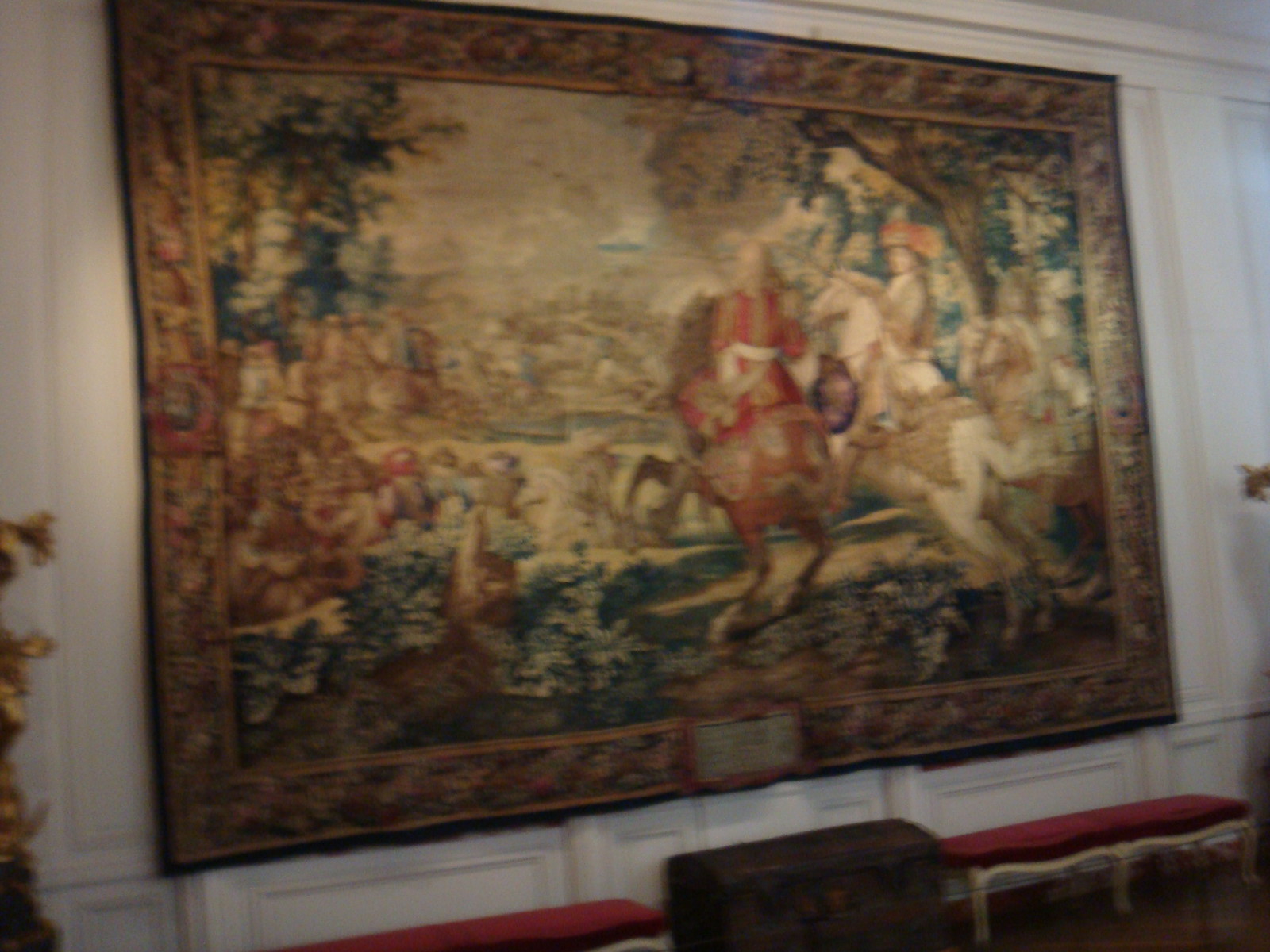The photograph captures a slightly blurry, angled image of an intricately designed tapestry or large area rug, hung on a white wainscoted wall. The tapestry depicts a detailed scene: at its center, a man in an old British military uniform of red with gold pauldrons and a white belt, rides a horse rearing up on its hind legs. To the right, there is a woman with long brown hair riding a white horse that has a brown saddle. On the left, various figures appear partly obscured by bushes, with one person notably kneeling on the ground. The far background reveals a cityscape of small white houses on a hill, set against a backdrop with additional horses. The tapestry is bordered by a floral print with a black edge and appears slightly wrinkled, as if not hung tightly. Below the tapestry, there are two white wooden benches with maroon cushions, and a trunk positioned between them at the bottom center of the photograph.